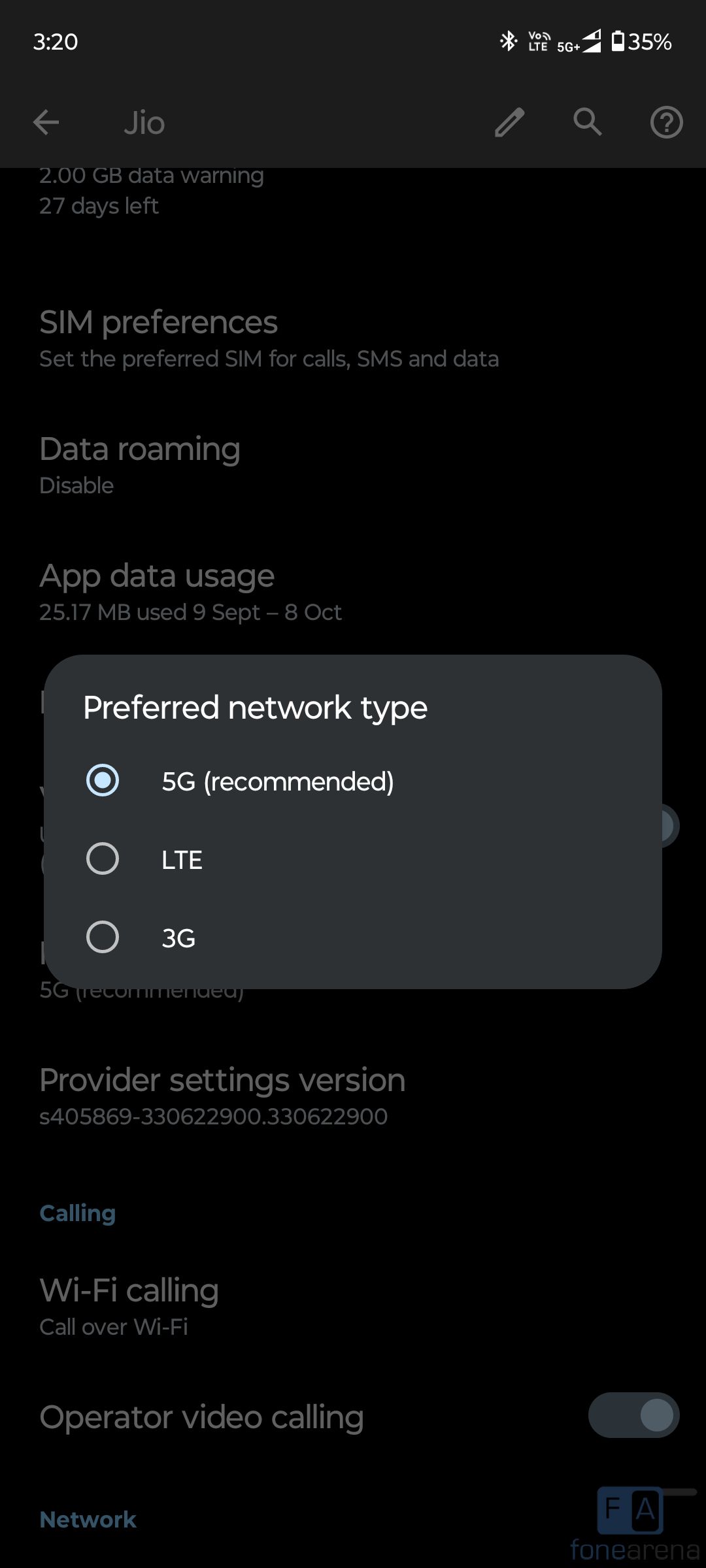The image is a screen capture of a cell phone's settings page, displayed on a black background with white text. The top left corner shows the time, 3:20. In the top right corner, there are indicators for Bluetooth, V-O-L-T-E, and 5G+ connectivity, along with two sets of Wi-Fi signal bars and a battery level reading at 35%.

At the very top of the screen, a slightly muted left arrow and the text "JIO" are visible. To the right, icons for a pencil, a magnifying glass (search), and an information question mark are lined up. 

Dominating the center of the image is a bright pop-up window titled "Preferred network type." Inside this pop-up are three radio buttons with options: "5G (recommended)," "LTE," and "3G." The "5G" option is selected.

Visible in the background, partially obscured by the pop-up window, are various sections and details including "SIM preferences," "Data roaming," "Operator video calling," "Wi-Fi calling," and "Provider settings." Additionally, it displays a version number and app data usage which states "25.17 MB used, 9 September - 8 October."